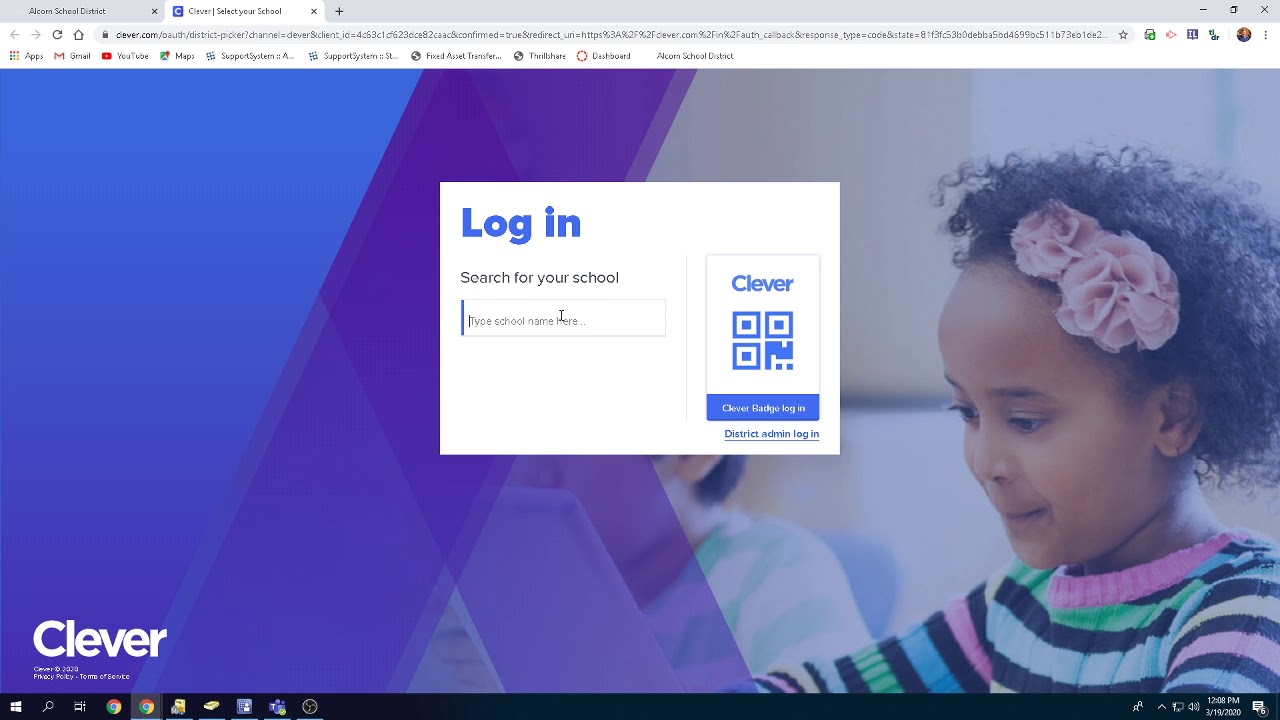The image showcases a login screen for a website, designed with a dual-color background predominantly featuring blue on the left side, interspersed with lines of purple. On the right side, an image of a joyful African-American girl wearing a multi-colored striped T-shirt in shades of blue, purple, and pink adds a lively and welcoming touch. Centrally positioned on the screen is a login notification prompting users to enter their credentials for website access. Beneath the login form, a prompt invites users to "search for your school," accompanied by a search bar for inputting queries. To the right of this section, a "Clever" branded QR code is visible, likely serving as an alternative login method. At the top of the browser, two open tabs suggest that the user is actively engaged with multiple web pages. The bottom of the screen displays the Google Chrome toolbar, featuring various icons for quick access to different applications and functions.